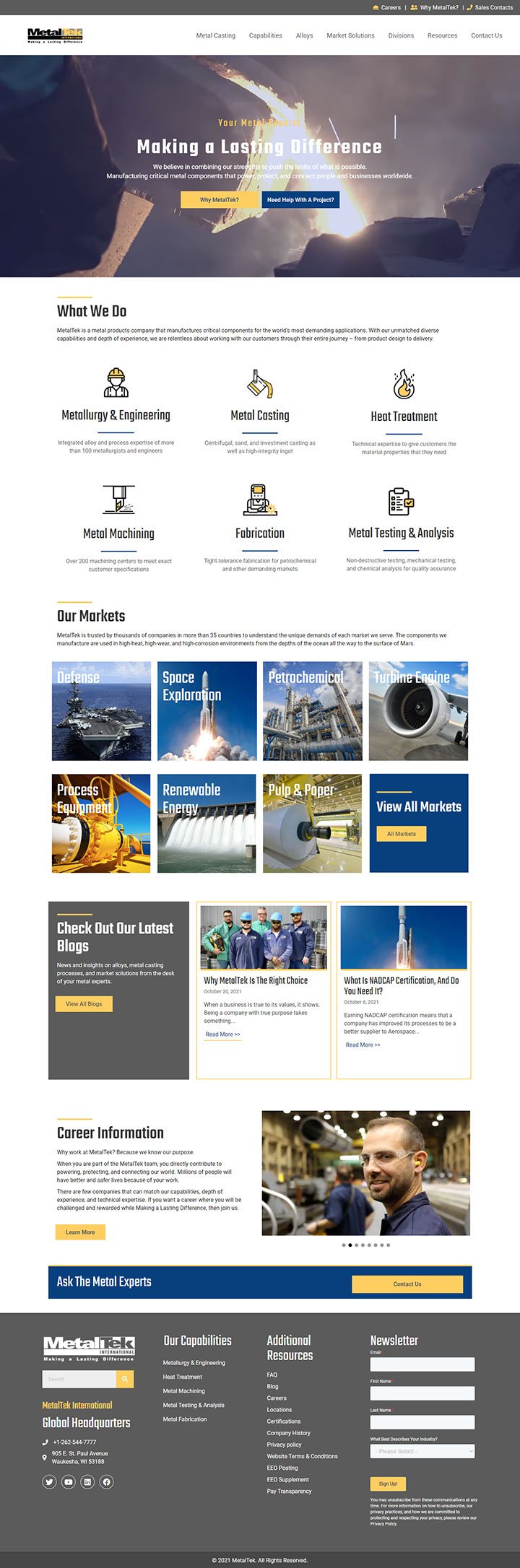The visual layout consists of multiple sections providing a detailed overview. 

At the top, a main rectangular banner prominently displays an image of a gray sky with a radiant yellow light at its center. Over this image, the motivational phrase "Making a Lasting Difference" is elegantly written in white text. Below this banner, in bold black text, the phrase "What We Do" introduces the next section.

This section lists various specializations in fine black text, highlighting key areas such as "Fabrication," "Metal Mechanisms," "Coding," and "Metal Casting," suggesting the company's expertise in construction and manufacturing services.

Further down, a grid of smaller squares features diverse images: a spaceship launching into space, the side of a contemporary white building, a large abstract yellow structure, and a man standing in front of a warehouse, looking at the camera with a slight smile, adding a personal touch.

At the bottom, a long blue rectangle houses a smaller yellow rectangular button, inviting viewers to click for more information.